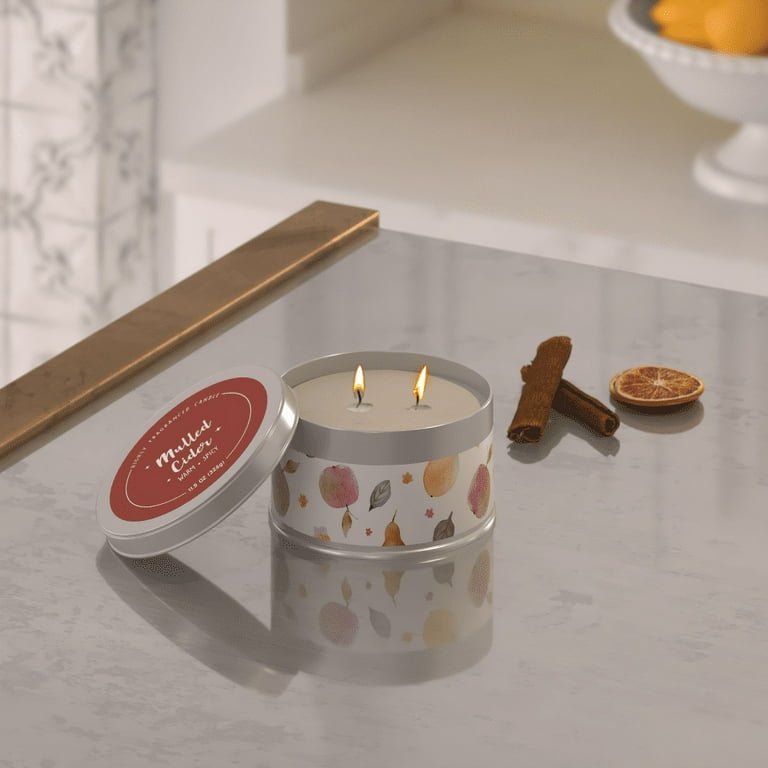In this image, a candle tin with a decorative label featuring colorful fruits such as apples, oranges, and possibly pears, sits centrally on a shiny silver table with a brown wood trim along the edges. The white wax inside the tin holds two black wicks, both lit, emitting a warm orange flame. The candle's lid, with a dark red label reading "mulled cider," lies off to the side. To the right of the candle, two cinnamon sticks and a dried orange slice are visible. The background details include a white-footed bowl with oranges on a white table and a wall adorned with black-and-white abstract floral wallpaper, adding depth and a cozy atmosphere to the scene.